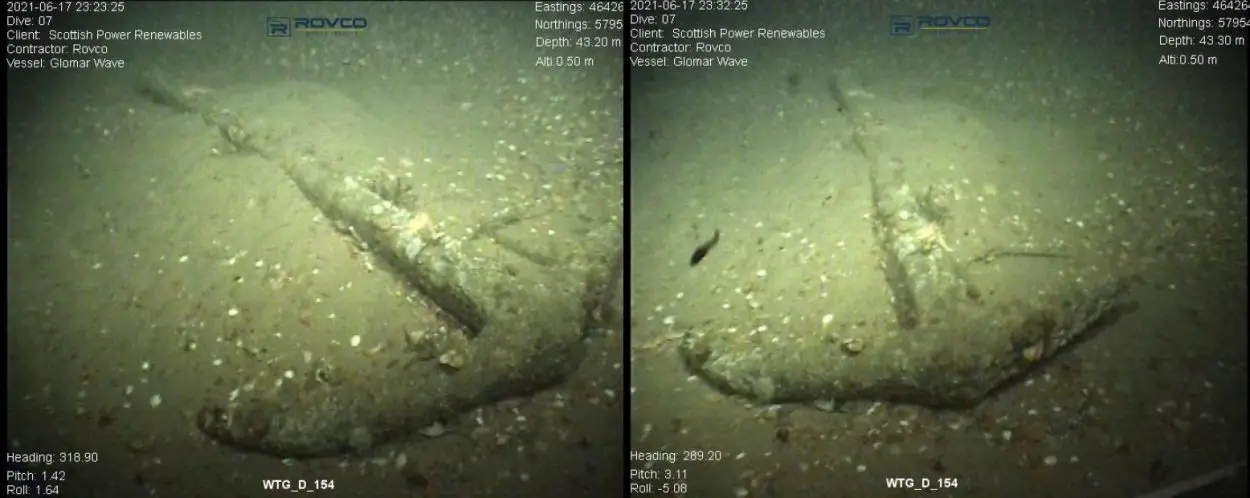This image showcases two side-by-side underwater photographs likely captured by a remotely operated vehicle (ROV) at the bottom of a body of water, possibly near a shipwreck. The murky, greenish water and low visibility suggest a significant depth. Both pictures depict what seems to be a large, partially buried boat anchor, surrounded by small rocks and bits of sea life, including a small black fish visible in the right image. The anchor's position varies slightly between the two angles. Above the photographs, there's detailed but small text including coordinates (Eastings 46426, Northings 5795), depth (43.2 meters), and other technical data. The date on the image reads 2021-06-17, with additional information about a dive (Dive 7) conducted by contractor Rovco for client Scottish Power Renewables, involving the vessel Glomar Wave. The company's logo, Rovco, is prominently featured on both images.